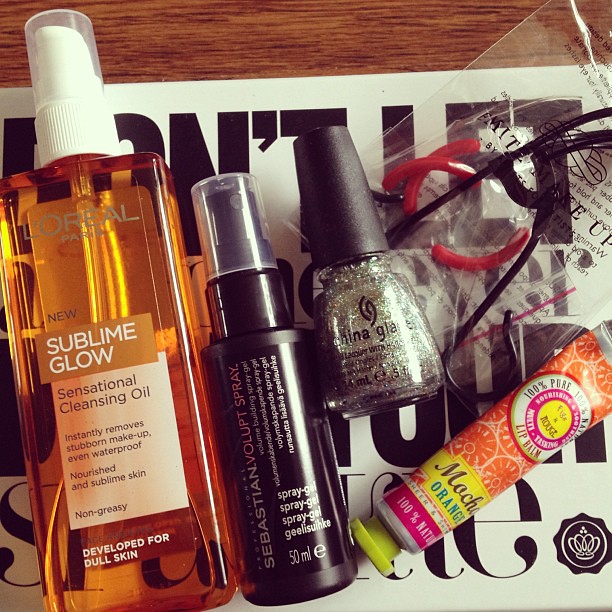The image depicts an assortment of beauty and makeup products neatly arranged on a wooden table indoors. Prominently displayed in the center is a white sign with black writing, possibly featuring motivational or promotional content. The products include an orange bottle from L'Oreal Paris labeled "New Sublime Glow Sensational Cleansing Oil," which promises to instantly remove stubborn makeup, even waterproof, while nourishing and revitalizing dull skin with a non-greasy finish. This bottle features a distinctive white spray cap. To the right of it sits a black spray gel by Sebastian, labeled "Volupte Spray Gel." Further to the right is a silver nail polish by a brand possibly named "Nina Glatt," with a chrome-like liquid inside. In the bottom right corner, there is a colorful tube of orange-scented lip balm, decorated with orange peel graphics and labeled "100% Natural." The table, acting as the backdrop, accentuates the carefully curated display of products.